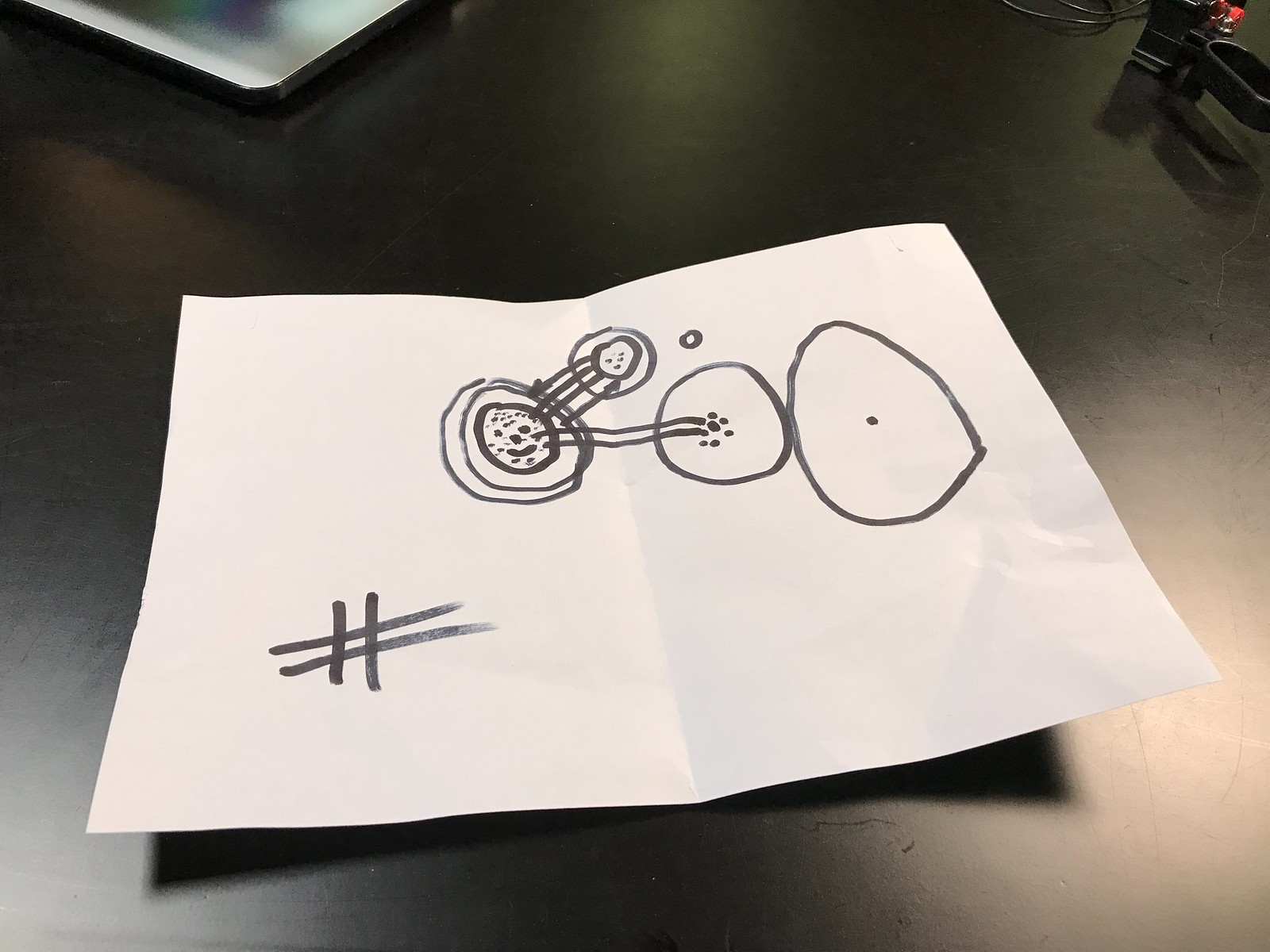This image depicts a photograph of a piece of paper placed on a black countertop. The black surface contrasts distinctly with the white paper in the foreground. 

In the image, the top right corner features an object with black and metallic criss-crossed wires, resembling a whisk. In the top left corner, there is a silver object. However, due to the angle or focus of the photograph, the details of these objects remain indiscernible.

Dominating the image is a white sheet of paper with a prominent crease down the middle, indicating it has been folded in half. The paper appears to hold a child's drawing, characterized by simple and whimsical shapes. In the bottom left corner of this drawing, there is a distinctive hash mark formed by intersecting lines.

The upper and central parts of the paper are adorned with a series of circles, varying in size and detail. The largest circle on the left contains a single dot in its center. Adjacent to it is a slightly smaller circle filled with numerous dots, connected to the previous circle by two wavy lines. Following this, there are two adjoining circles, featuring a smiley face in their center. Further wavy lines extend from the smiley face to another structure, a circle within a circle, also filled with dots. Additionally, arrows are drawn pointing towards and away from the smiley face, indicating movement or a flow between the shapes.